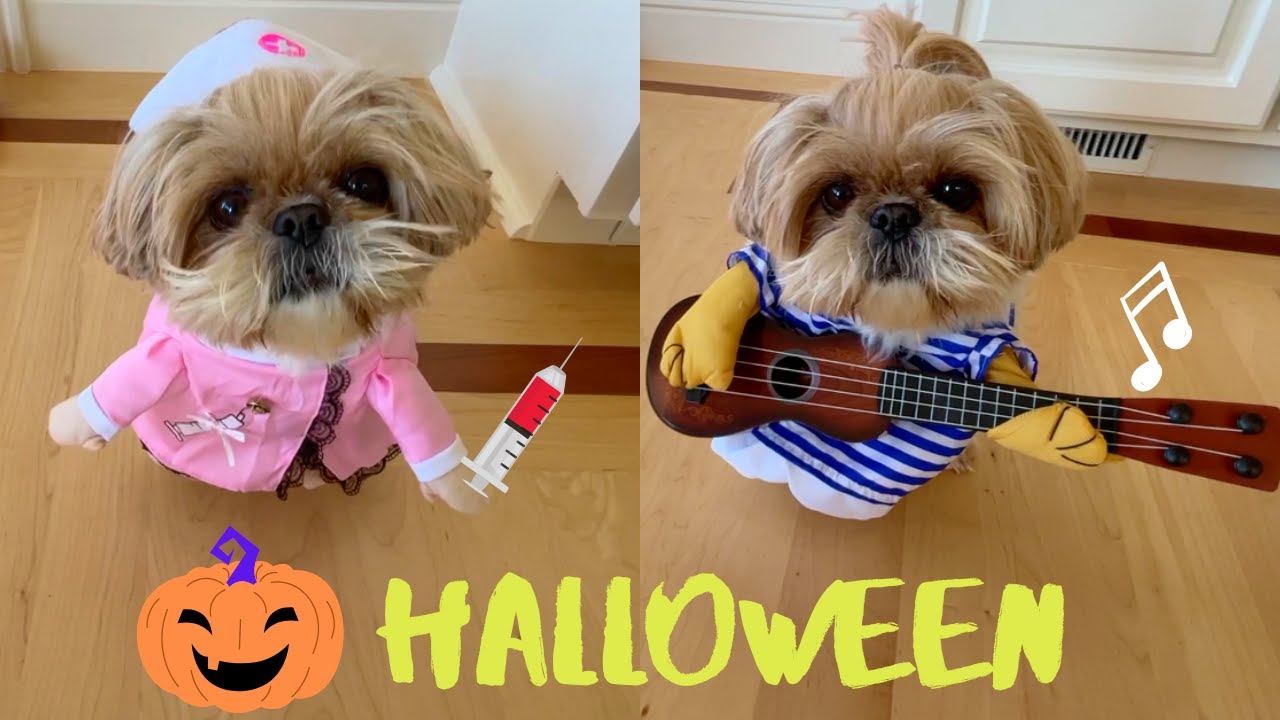This is a set of side-by-side, indoor photos of the same small, sandy brown dog, possibly a Shih Tzu or Lhasa Apso, dressed in two different Halloween costumes. The left photo features the dog in a pink nurse outfit complete with a nurse's cap, a blue top with white cuffs, and a syringe in one of the attached hands. The right photo shows the dog dressed as a musician, with its top fur pulled up with a rubber band and wearing an outfit with gray, blue, and white stripes, holding a guitar or ukulele. The bottom part of the image features a computer-generated Halloween graphic, including a pumpkin and the word "Halloween" in a spooky font. The photos appear to be superimposed on a wooden floor background. The right image also has a musical note above the dog, enhancing the musician theme.